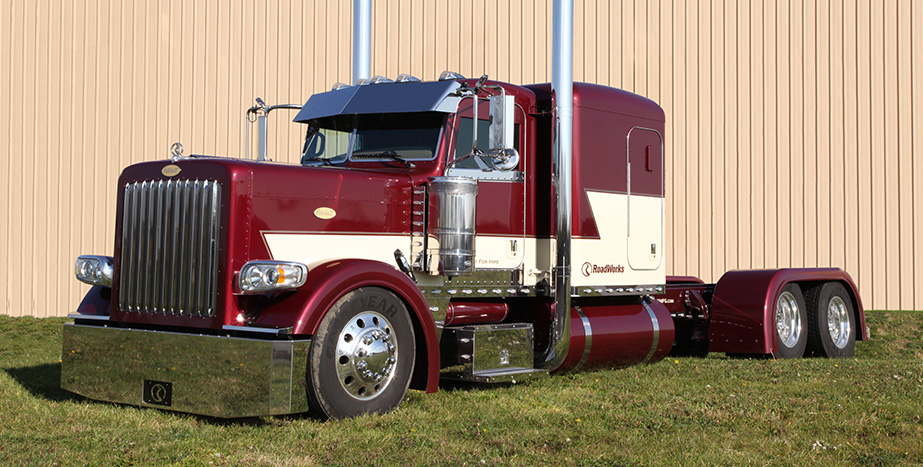The outdoor image showcases a pristine, glossy burgundy Kenworth semi-truck without a trailer, parked on a field of short green grass in front of a large building. The building features vertically aligned, tan-colored, corrugated metal siding. The truck, seemingly a showpiece given its immaculate condition, boasts a massive sleeper cab and is accentuated with extensive chrome detailing. A cream-colored stripe zigs and zags up the sleeper cab, contrasting elegantly with the burgundy body. The front bumper and grill are exceptionally shiny and reflect the surrounding grass. Two towering silver smoke stacks rise up from either side of the truck, complementing other chrome elements like the visor around the front window, wheel covers, steps, mirrors, and a variety of other chrome accents. Despite the impressive details, no people are visible inside the darkened cab.